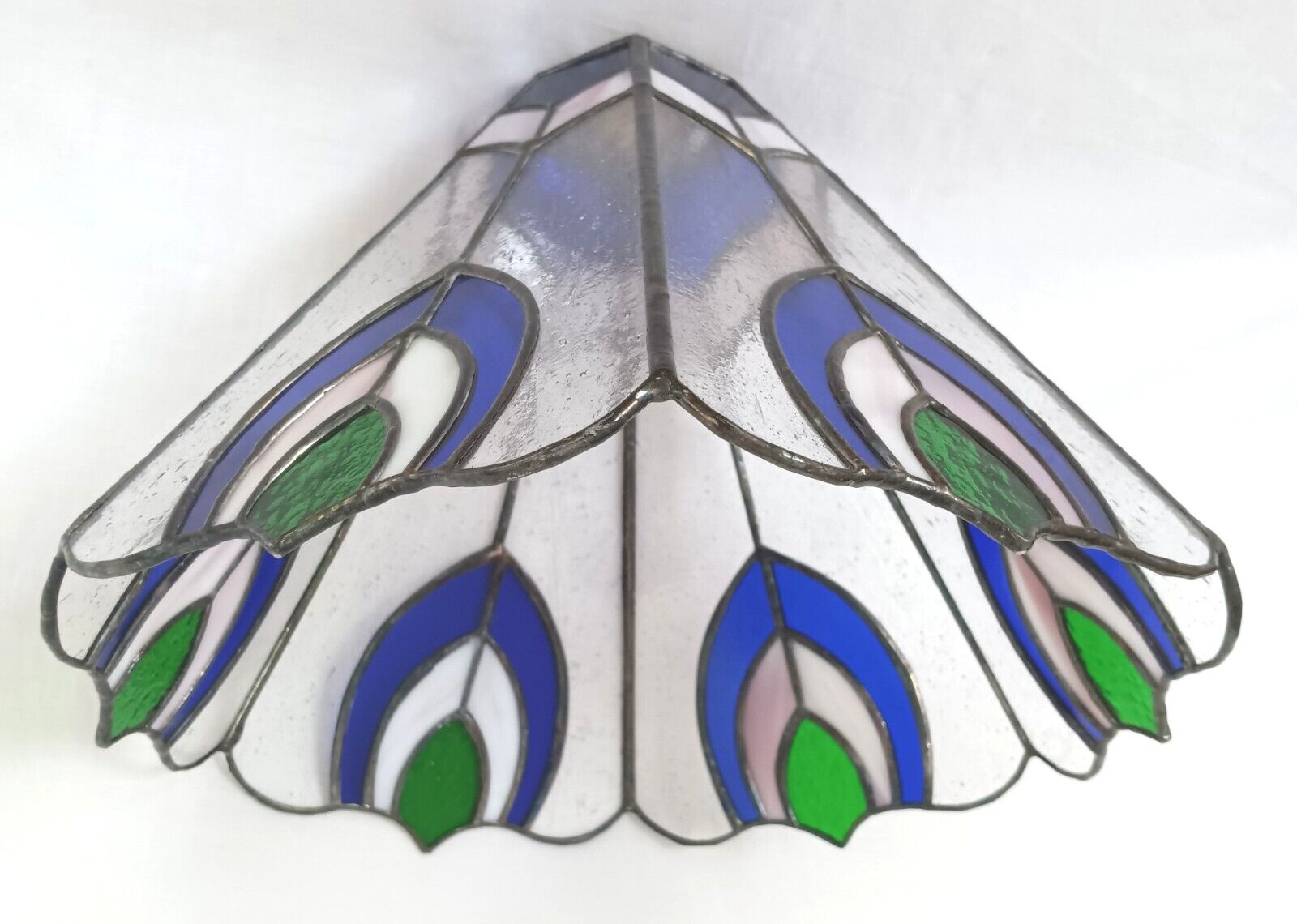The image showcases a glass lampshade captured from a bottom-up perspective, emphasizing its intricate and colorful details. The lampshade adopts a diamond-like shape and features a hollow bottom, with a series of painted half-circle patterns adorning its inner bottom surface. The bottommost half-circle is blue, followed by a white one, and then a green half-circle, giving it a layered appearance. The glass is predominantly white inside but has translucent properties, slightly blurring the view through it. Notably, there's a blue upside-down U-shape near the edge, housing a green leaf-like design within it. The top of the lampshade is black with a light black border encircling the blue design, adding contrast to the translucency of the glass. The background of the image is white, further highlighting the detailed patterns and colors of the lampshade.